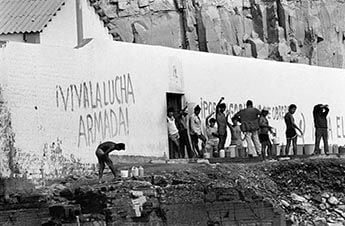In this striking black-and-white photograph, a large group of protesters is gathered in front of a prominent white wall. The image, devoid of color, emphasizes the stark contrasts and adds a historic feel, suggesting it dates from the past. The protesters, raising their fists in a display of solidarity and resistance, seem to embody the spirit of revolution. Behind them, the wall is adorned with revolutionary slogans, including the bold phrase "Viva La Lucha Armada" (Long Live the Armed Fight). The wall stands in front of an old house partially visible, and the scene is set against a rugged, mountainous backdrop. To the side, a rocky hillside strewn with debris slopes downward, enhancing the sense of a tumultuous, possibly quarry-like environment. The photograph captures a moment charged with tension and defiance, framed by a landscape as severe and unyielding as the protesters' cause.